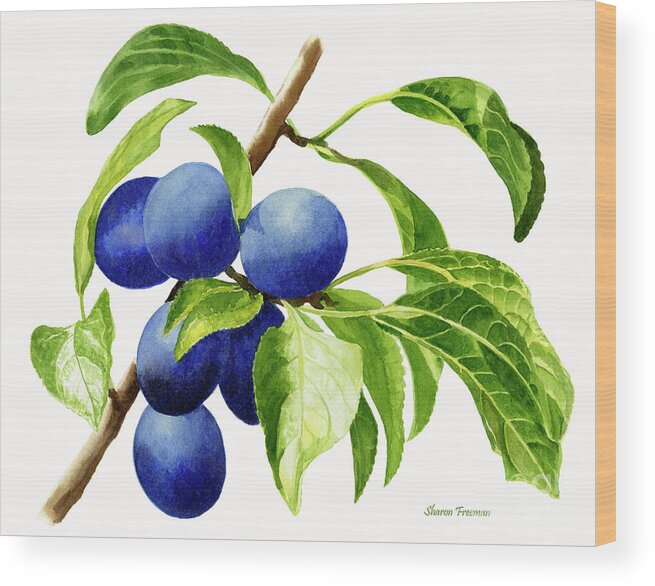This image features a detailed painting on a slightly angled, white canvas about an inch or two thick. The right-hand side reveals a wooden edge beneath the canvas. The painting itself depicts a delicate, thin brown branch extending diagonally from the bottom left to the top middle of the canvas. Attached to the branch are several green leaves and a cluster of strikingly blue, round grapes, arranged with three in a row, two below, and one more beneath them. The blue hue of the grapes, which stand out vividly, might also suggest they could be blueberries. The bottom right corner of the artwork features the artist's signature, "Sharon Freeman," written in elegant script. The clean and visually appealing composition showcases the natural elements of the branch and fruit, making it a standout piece.